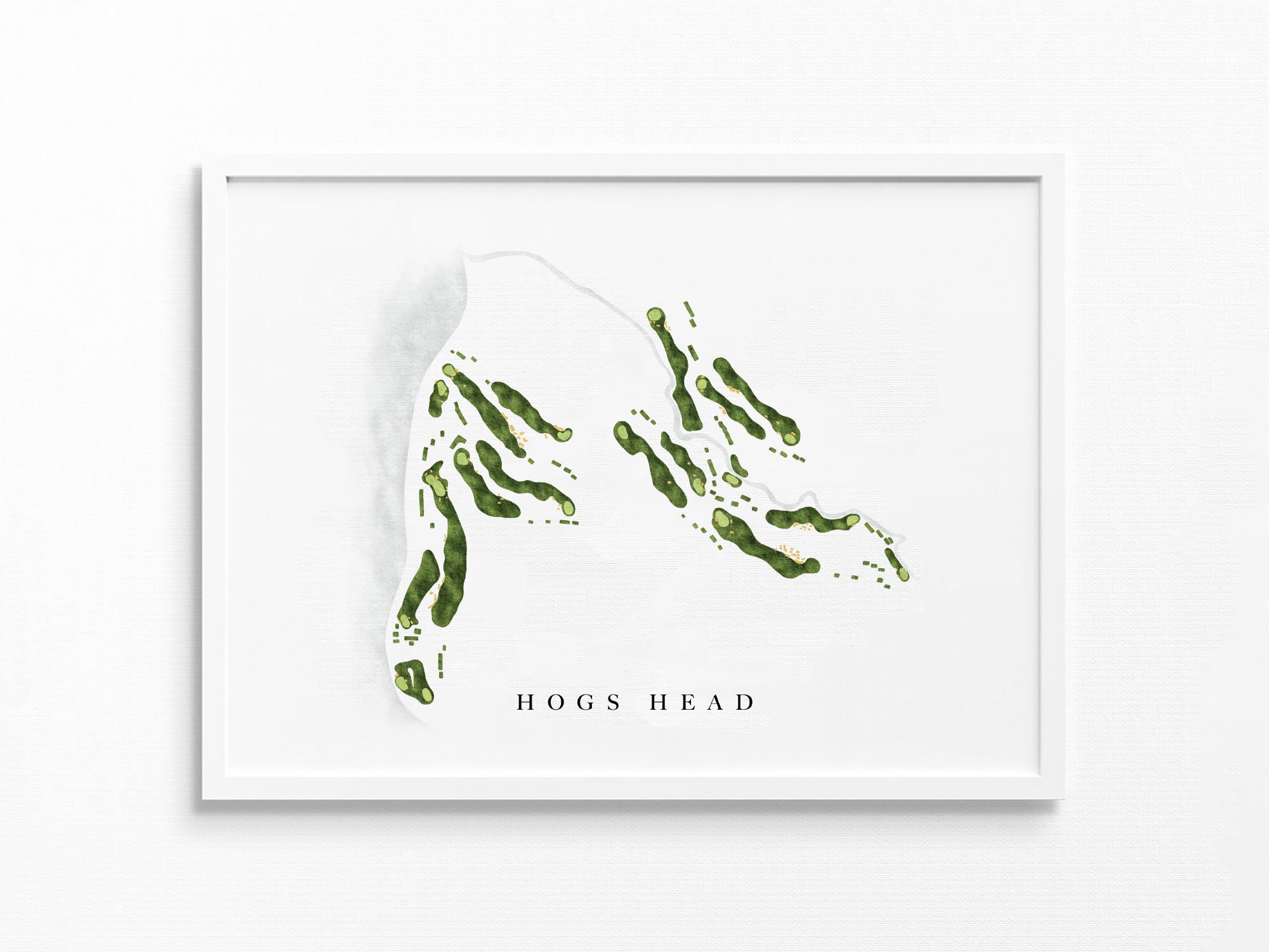In this image, we see a color photograph of a framed piece of artwork displayed on a white wall. The artwork, surrounded by a pure white frame, features a predominantly white canvas as its backdrop. Central to the composition are several green, tube-like shapes resembling string beans or worm-like forms, each with lighter green tips. These shapes appear to be swimming or floating upwards toward the top left corner, leaving behind small, dotted green trails. A subtle shadow is cast to the left of these green forms. At the bottom of the image, the text "HOGS HEAD" is prominently displayed in black, all-capital letters, separated into two words. The artwork's arrangement of green shapes is irregular and unpatterned, adding a dynamic feel to the minimalist piece.